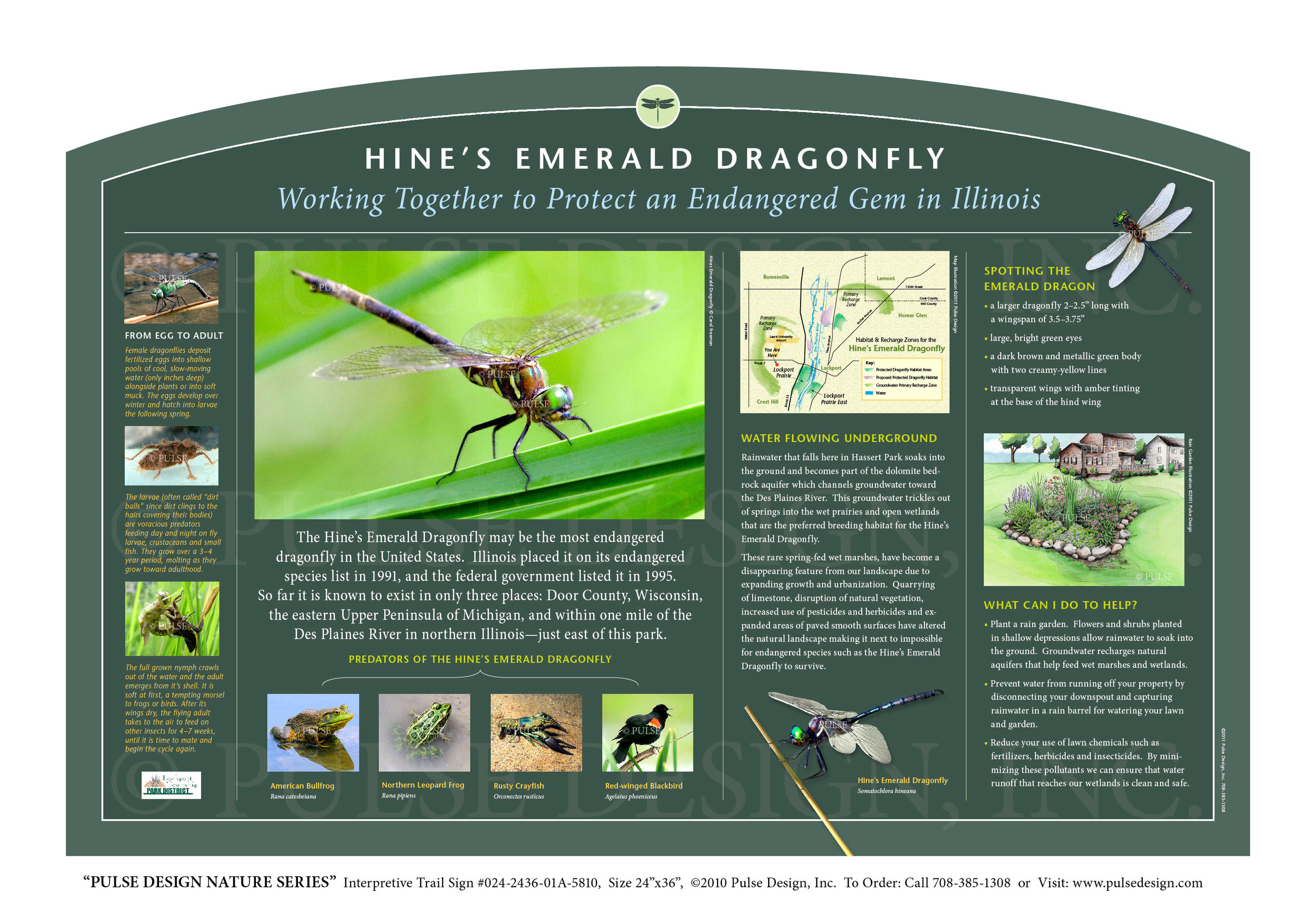This flyer is dedicated to raising awareness about the Heinz Emerald Dragonfly, an endangered species in Illinois. The flyer features a dual-toned green design, with a light green border and a darker green center. Prominently displayed in white lettering is the headline, "Heinz Emerald Dragonfly," followed by green lettering: "Working together to protect an endangered gem in Illinois."

The flyer includes various images related to the dragonfly, the most striking of which is a larger picture of a dragonfly perched on a leaf, its wings spread wide. Additional visuals include a smaller dragonfly in flight, as well as photos illustrating the dragonfly's life stages from egg to adult. The imagery is complemented by pictures of its natural predators, such as birds and a bullfrog.

The main text highlights the endangered status of the Heinz Emerald Dragonfly, noting it is one of the most endangered dragonflies in the United States. Illinois recognized the species as endangered in 1991, with federal recognition following in 1995. The species is currently known to exist in only three locations: Door County, Wisconsin; the eastern upper peninsula of Michigan; and within one mile of the Des Plaines River in northern Illinois.

The flyer also includes sections like "Spotting the Emerald Dragonfly," "Water Flowing Underground," and "What Can I Do to Help?" to engage readers in conservation efforts. The design is part of the Pulse Design Nature Series.